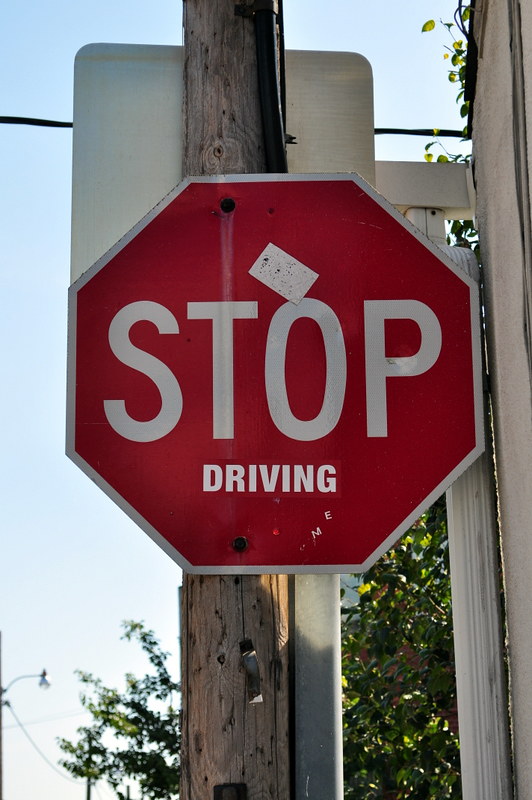This color photograph, taken on a clear, sunny day, features an altered American stop sign prominently centered in the image. The standard octagonal stop sign, with its familiar red background, white outline, and "STOP" in bold white capital letters, has been modified. Beneath the word "STOP," a sticker with a matching red background and white letters spells out "DRIVING," making the sign read "STOP DRIVING." Additionally, a small white rectangular sticker, akin to a half-width sticky note, is diagonally placed above the "O" in "STOP," slanted towards the right.

The stop sign is mounted on a vertically oriented wooden utility pole that stretches from the bottom to the top of the frame. The pole also supports another street sign on its opposite side, only part of which is visible—the back of a tall vertical rectangular sign. The backdrop includes a light blue sky without clouds, green trees on either side of the pole, and a tan fence or wall partially visible in the right of the frame. Additionally, a black utility line runs horizontally across the upper part of the image, partially concealed by the signs and pole.